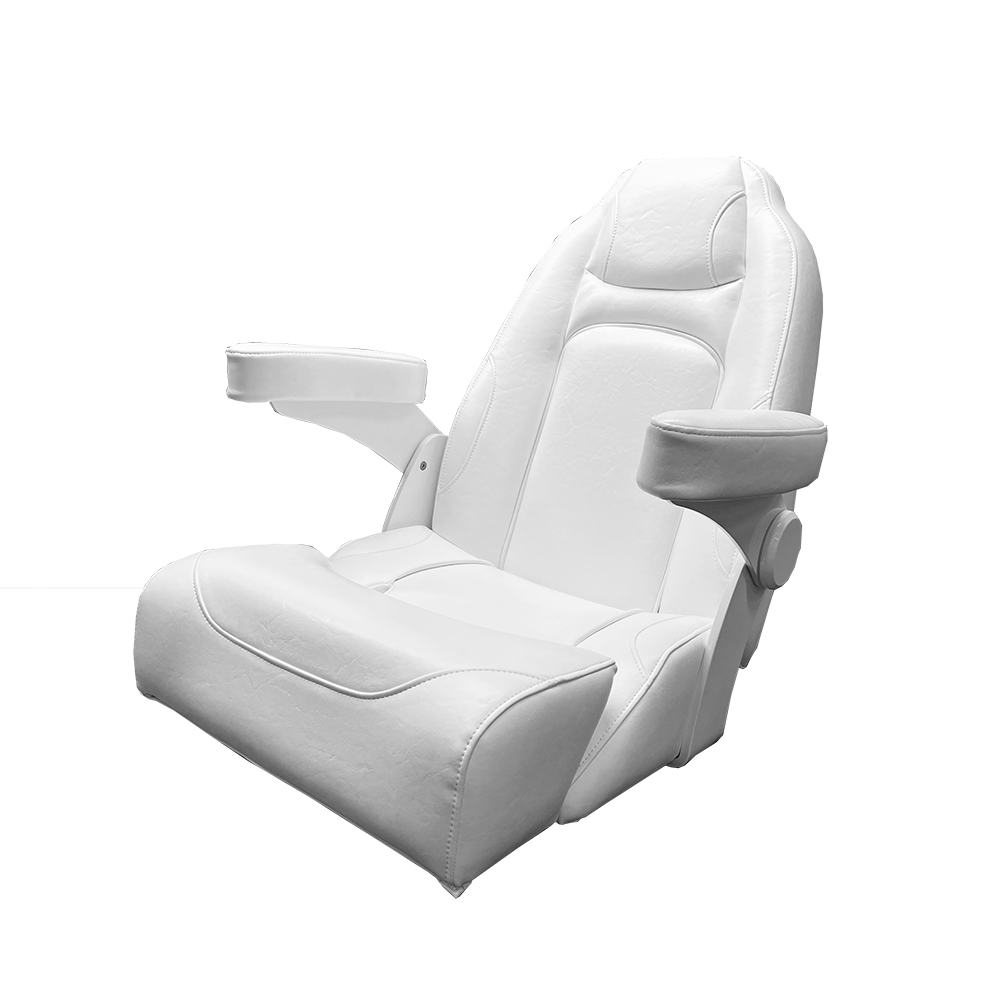This image showcases a high-back, all-white leather-like chair, likely designed for a premium setting such as a plane, bus, or movie theater. The chair exhibits an elegant and ergonomic design. The backrest features a distinctive round hump, a central section, and a headrest accented with two stitching marks on both sides, providing excellent support. Attached to the headrest are shoulder pad supports that complete the upper section of the chair. The seat itself is split into two stitched sections for enhanced leg and rear comfort. The armrests are supported by plastic frames connected with screws and include padded tops with a stitched pattern for forearm support. The chair lacks visible legs, suggesting it is intended to be mounted in a fixed location, contributing to its refined and streamlined appearance. The entire backdrop is white, emphasizing the chair's pure and sophisticated aesthetic.